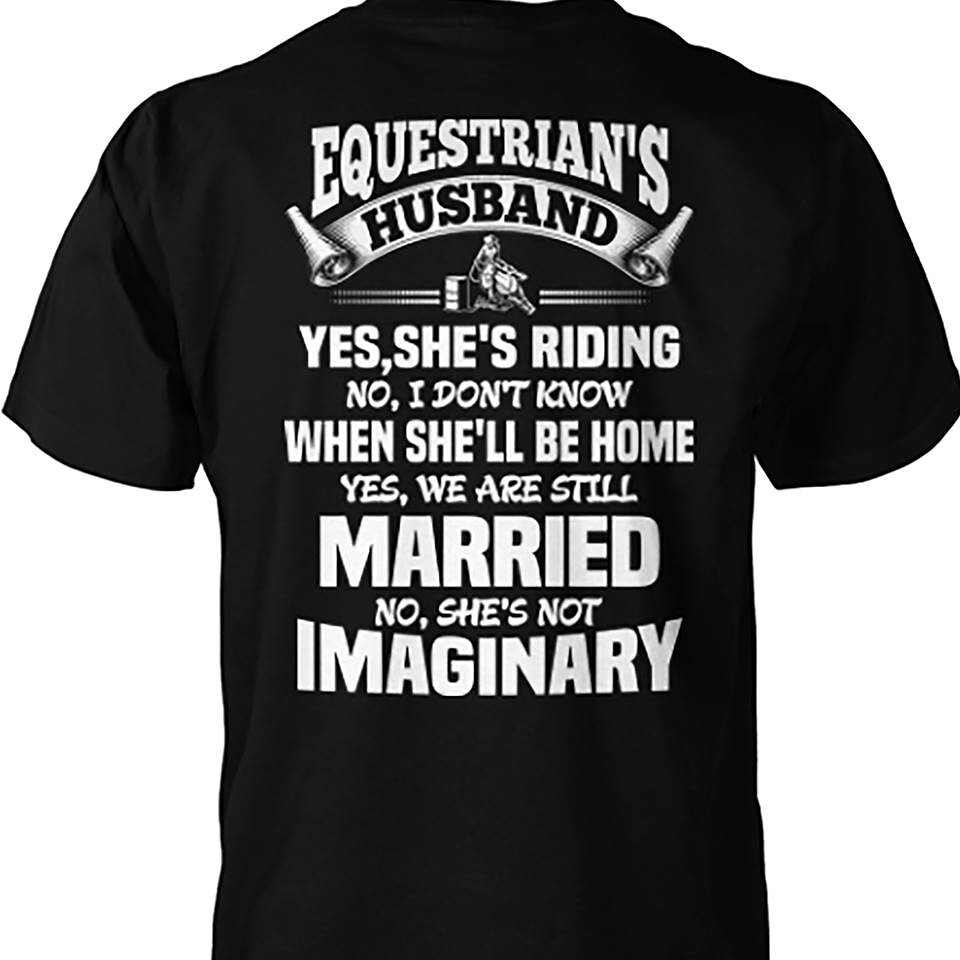The image depicts the back of a black t-shirt presented against a white background, emphasizing a humorous and detailed text graphic in white. At the top, the text reads "Equestrian's Husband" with "Husband" curated on a scroll banner. Below this banner, there is a graphic of a woman riding a horse, resembling a jockey or equestrian figure. Underneath the image, bold block capital text reads, "YES, SHE'S RIDING," followed by the line "NO, I DON'T KNOW WHEN SHE'LL BE HOME." The text continues with "YES, WE ARE STILL MARRIED," and concludes humorously with "NO, SHE'S NOT IMAGINARY." The typographic design utilizes various fonts and layout styles, with the words "MARRIED" and "HUSBAND" prominently highlighted in bold, adding contrast and emphasis. The t-shirt displays elements of silver-ish detailing on the scroll and horse graphic, and the overall design evokes a blend of product photography realism.